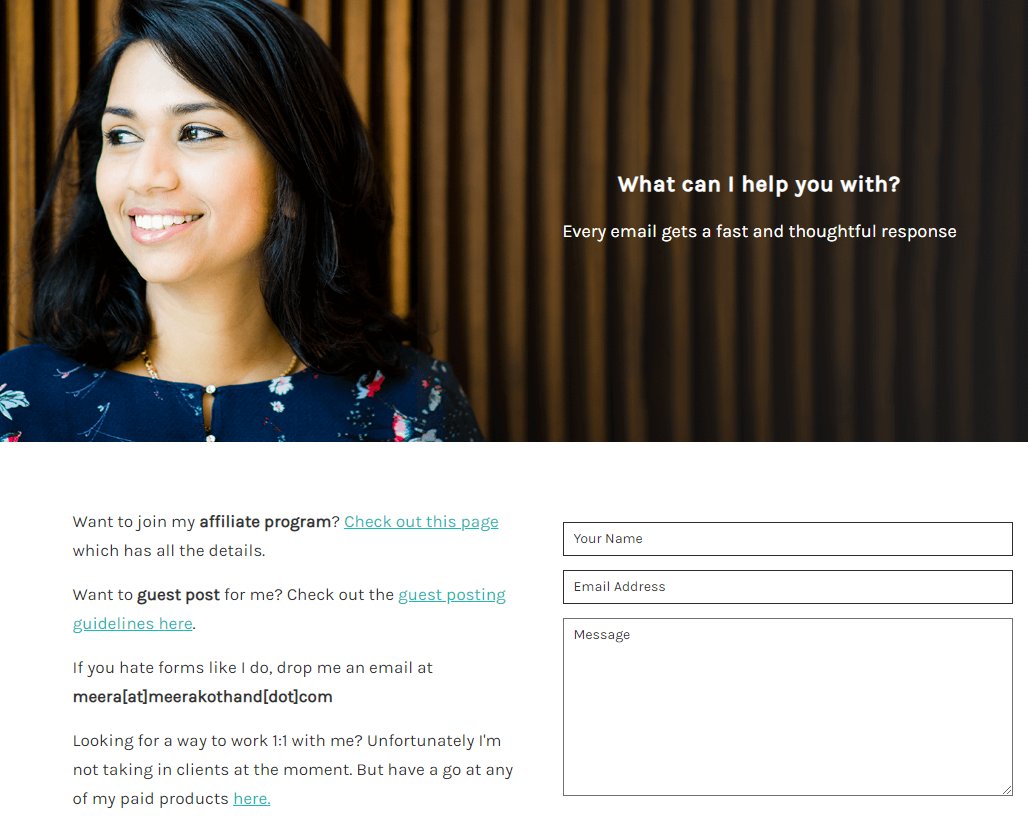The image captures a web page featuring a woman with dark black hair, smiling as she gazes off to the left. She wears a gold necklace and a dark navy dress adorned with lighter-colored floral patterns. She stands against a brownish wall, and across this wall in white print is the text, "What can I help you with?" Below this, smaller print reads, "Every email gets a fast and thoughtful response."

At the bottom left of the page, there's an invitation: "Want to join my affiliate program?" followed by a blue link stating, "Check out this page," and returning to black text, "which has all the details."

Further down, the page prompts, "Want to guest post for me? Check out the," with an underlined link continuing, "guestpostingguidelines.here."

Beneath this, the text reads, "If you hate forms like I do, drop me an email at," followed by her email address. It then continues, "Looking for a way to work one-on-one with me? Unfortunately, I'm not taking any clients at the moment, but have a go at any of my paid products here," with the phrase "paid products" presented as a blue link.

At the bottom of the webpage are three input fields for name, email address, and message, inviting visitors to get in touch directly.